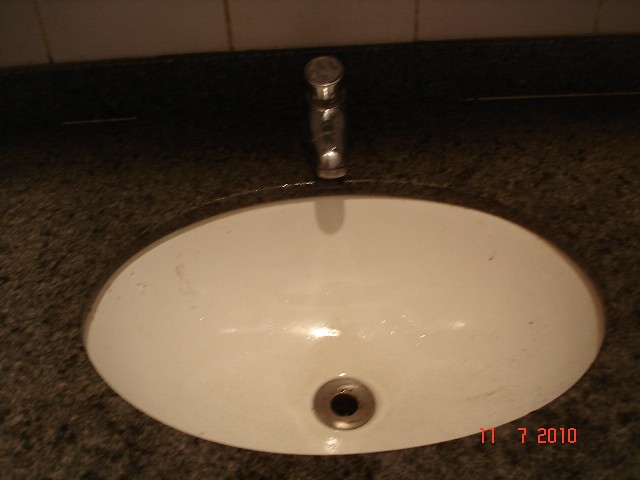This photograph, dated November 7, 2010, showcases a bathroom sink set against a backdrop of brown wooden paneling. The basin, slightly dingy and off-white, exhibits subtle striations or cracks, adding character to its surface. It is encased in a countertop that mimics the appearance of black or brownish-black marble. The sink features a chrome faucet with a single handle for water adjustment, indicative of a design that lacks visible hot or cold indicators. The drain is surrounded by a silver, slightly brassy ring, leading to a dark, shadowed central hole. The image is dimly lit, casting shadows that accentuate the textures and surfaces, with the only text being the bright red date stamp.